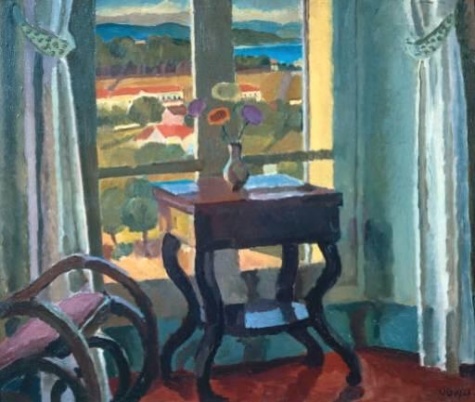This still life impressionist painting, possibly watercolor or oil-based, captures an indoor scene of a cozy room with a prominent window overlooking a serene countryside. The window is adorned with white drapes on either side and partially blocked at the bottom by a brown desk with black legs. Centered on the desk is a vase containing four flowers: two violet, one yellow, and one red. To the left of the desk, a brown-legged rocking chair is partially visible. 

Through the large window, the expansive view reveals lush green trees in the foreground, a blue lake or river in the middle distance, and a majestic range of mountains under a sky dotted with clouds on the horizon. The room features a red carpet and possibly blue walls, with a dark blue corner marking the junction between floor and walls, which adds depth to the painting. The color palette includes prominent blues and whites, enhancing the tranquility of the scene. There is also an indistinct painter's signature subtly included within the artwork, adding a touch of authenticity. Overall, the painting beautifully harmonizes an inviting indoor setting with a picturesque countryside vista, rendering a peaceful daytime depiction.